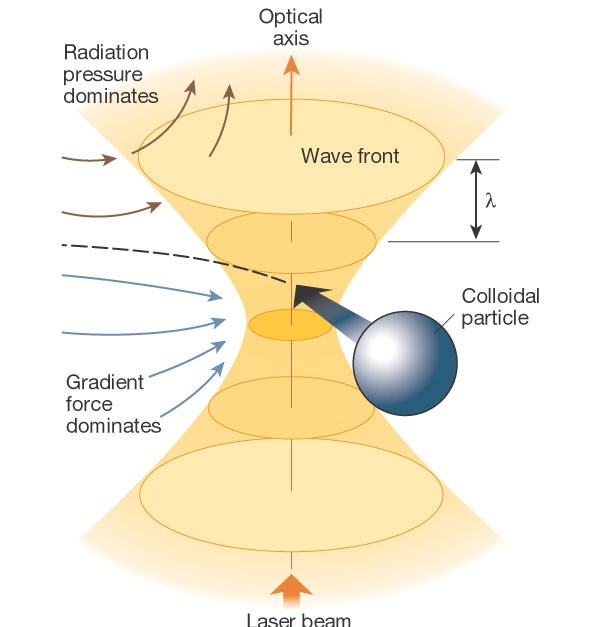The image is a detailed science diagram resembling those found in physics textbooks. It prominently features a yellow, hourglass-shaped cylinder constricted in the middle, suggestive of a wave or beam. Various arrows in colors like orange, dark red, and blue point towards and away from the cylinder, each annotated with specific text. At the center, a dark blue arrow intersects a dark blue circle labeled "colloidal particle." Additional arrows at the bottom and top of the diagram are labeled "laser beam" and "optical axis," respectively. The diagram also contains text indicating where "radiation pressure dominates" and "gradient force dominates," illustrating fundamental principles of physics related to particle behavior and laser interactions. The overall layout and intricate labeling suggest it explains the functioning of a particle collider or a related scientific apparatus involving lasers and colloidal particles.